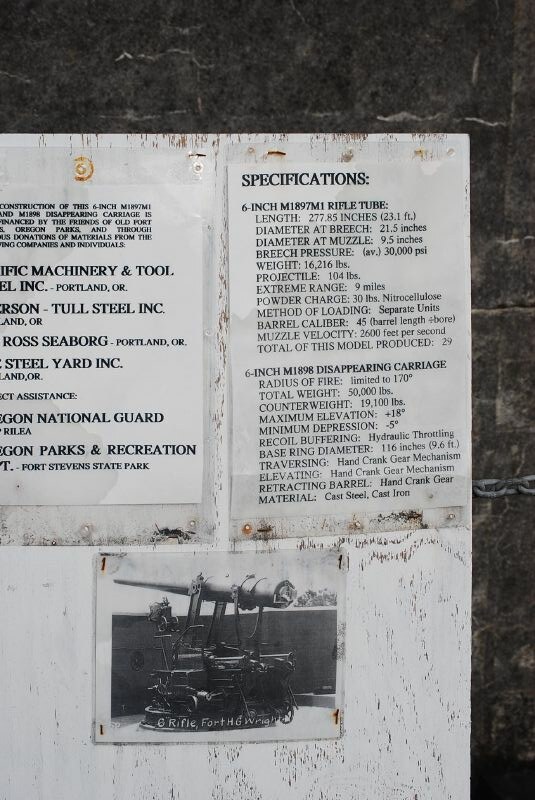This image depicts an old, weathered piece of wood painted white, with the paint partially peeled away to reveal the grain underneath. Affixed to the wood is an ancient-looking piece of paper, displaying detailed specifications in black and white. The background features a dark, stone wall and a chain. The specifications detail a 6-inch M1897M1 rifle, including its dimensions, weight, and loading method. A black-and-white illustration of the rifle is present on the bottom of the paper, providing a visual reference of the weapon.